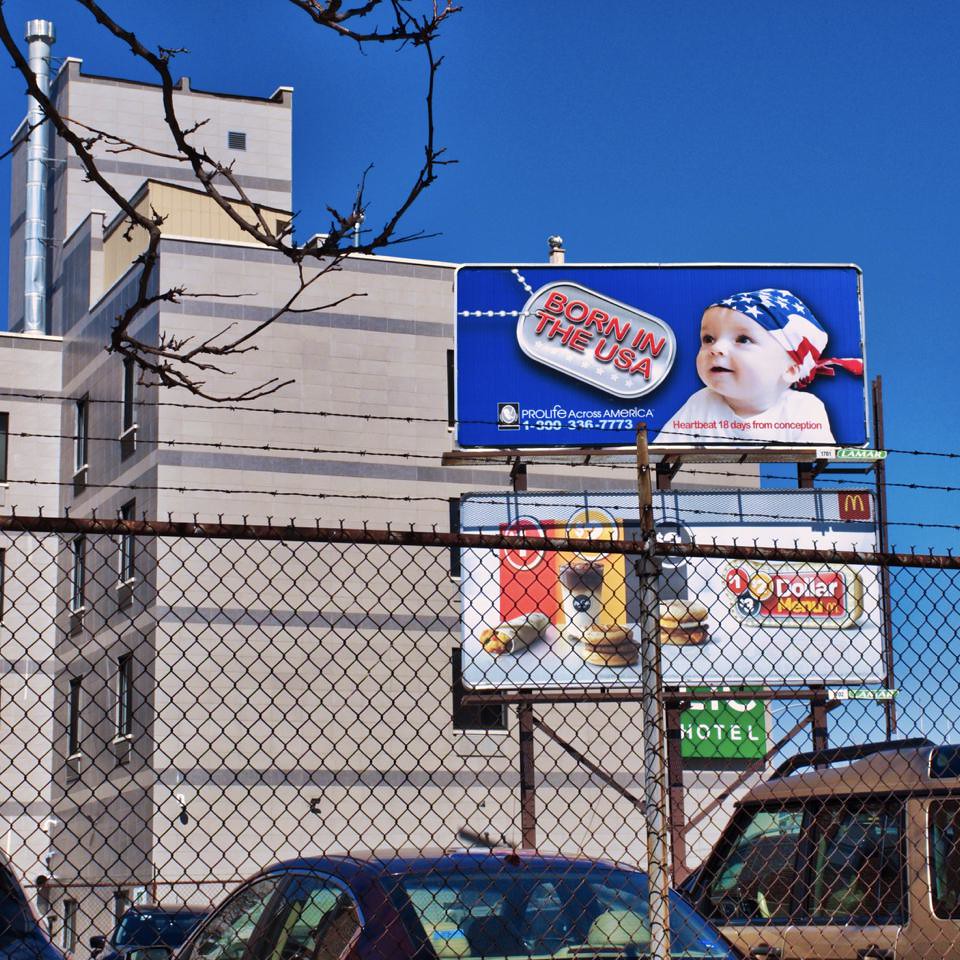A daytime photograph captures two billboards positioned in front of a gray building, framed by chain-link fences on either side. In the foreground, a parking lot is partially visible, with several cars scattered around. A clear blue sky stretches above, and tree branches intrude slightly into the frame from one quarter of the image.

The top billboard features a patriotic design, displaying a pair of dog tags with the words "Born in the USA" in bold red font against a blue background. An infant wearing a white shirt and an American flag-themed head covering is prominently featured on the billboard.

Beneath this, a second billboard advertises McDonald's Dollar Menu. The iconic McDonald's logo is visible in one corner, while the rest of the billboard showcases tantalizing images of a breakfast burrito and two breakfast sandwiches, enticing viewers with affordable morning meal options.